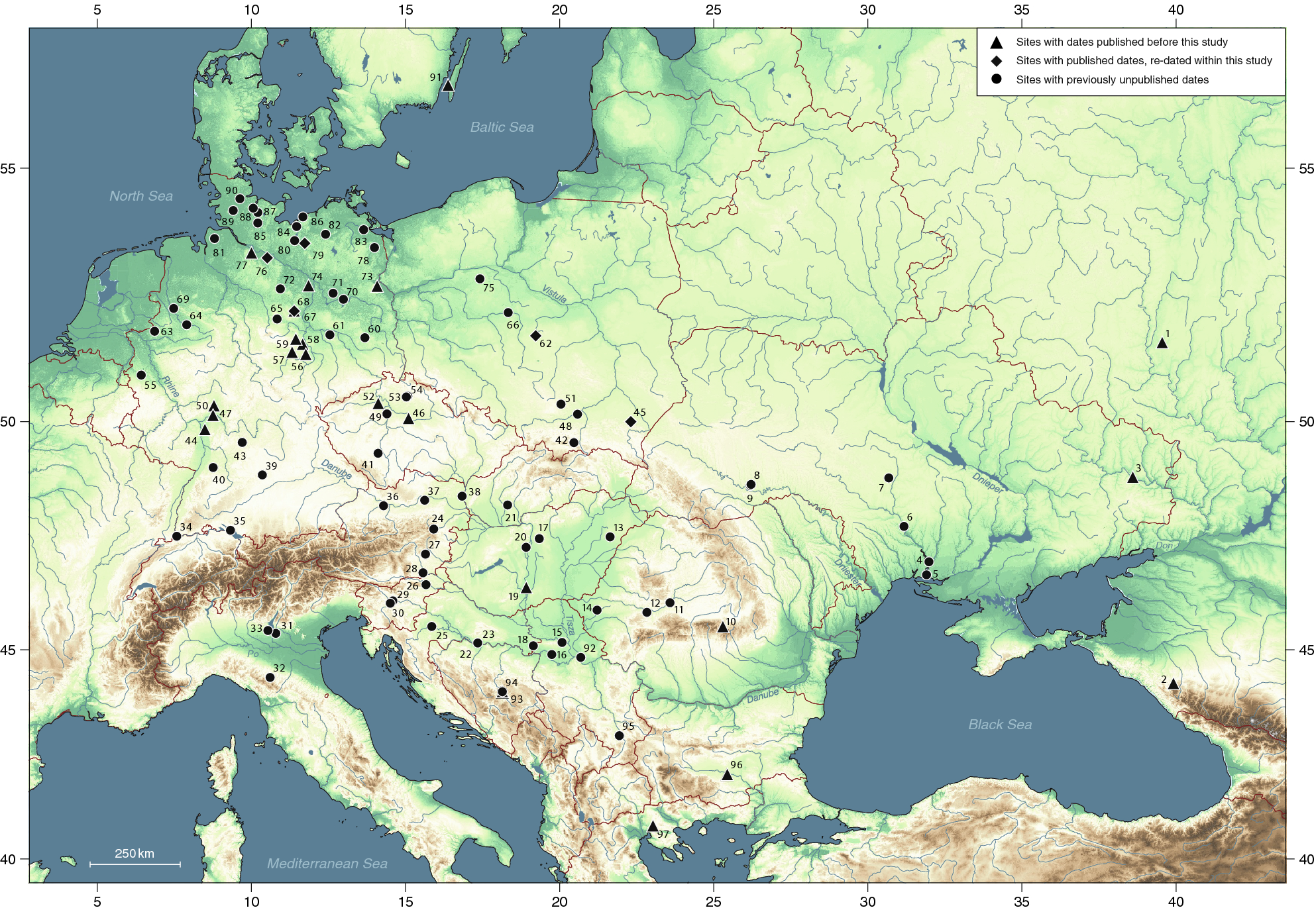The image is a detailed map predominantly depicting Europe and extending into parts of Asia. Although the countries are unnamed, the surrounding seas are clearly labeled: the Baltic Sea in the north, the North Sea to the northwest, the Mediterranean Sea in the south, and the Black Sea in the southeast. The map features various symbols, including triangles, diamonds, and circles, each accompanied by numbers. The legend, located in the top right corner, clarifies that triangles represent states with data published before the study, diamonds denote states with published dates redated within the study, and circles indicate sites with previously unpublished dates. Additionally, a scale in the bottom left shows a measurement of 250 kilometers. The map includes a mix of colors like green, red, brown, and white, enriching its detailed depiction of the region’s geography and data points.